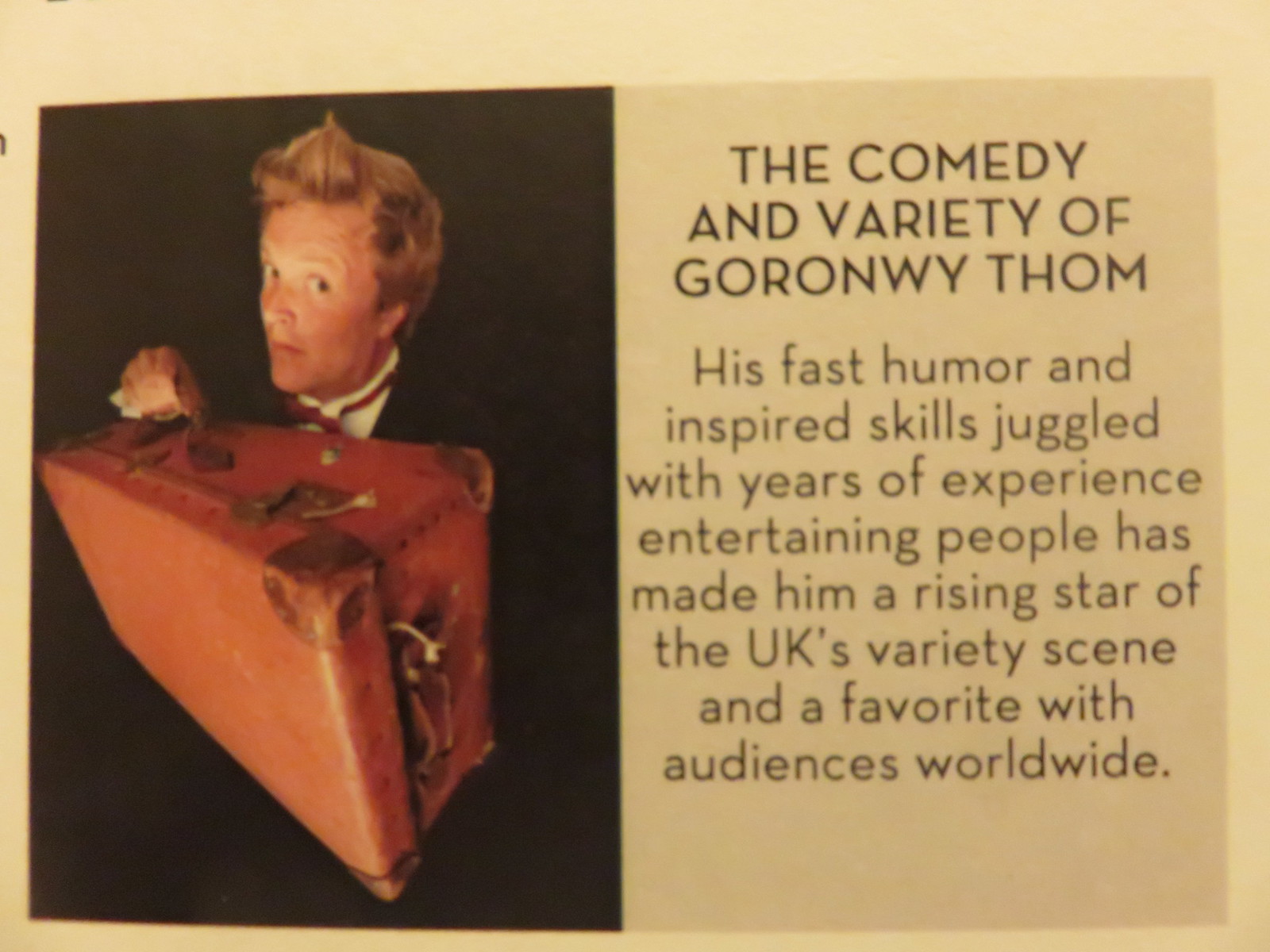The image features a striking split design with the left side dominating a black backdrop, showcasing a man from the chin up. He possesses reddish blonde hair and no facial hair, his expression marked by raised eyebrows and a side-eye glance, adding a touch of intrigue. This man, clad in a black suit coat and white collared shirt, is distinguished by a red bow tie peeking out. Held up in his right hand and angled toward the camera is an old-fashioned, hard, dark brown briefcase with orangey undertones. The right side contrasts sharply with a vibrant yellow background and black text, promoting "The Comedy and Variety of Goronwy Thaum." The text extols his fast humor and inspired skills, honed over years of experience, making him a rising star in the UK's variety scene and a beloved figure among audiences worldwide.